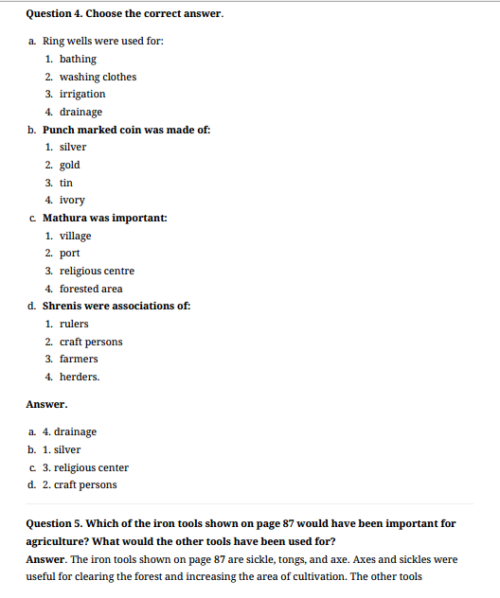A detailed and cleaned-up description of the image could be:

---

The image is a black and white photograph of a text-based document, devoid of any images. At the very top of the page is a gray line. Directly below this line, in bold text at the top left corner, it states "Question Four: Choose the correct answer." The document proceeds with a series of multiple-choice questions.

- **Question A:** To the left is the letter "A" and to the right, the question reads, "Ring wells were used for:" followed by the choices:
  1. Bathing
  2. Washing clothes
  3. Irrigation
  4. Drainage

- **Question B:** The letter "B" is accompanied by, "Punch mark coin was made of:" with the options:
  - Silver
  - Gold
  - Tin
  - Ivory

- **Question C:** Following with "Mathura was an important:" the choices listed are:
  - Village
  - Port
  - Religious center
  - Forested area

- **Question D:** The letter "D" is followed by, "Shrenas were associations of:" and the options are:
  - Rulers
  - Craftspersons
  - Farmers
  - Herders

At the bottom of the list, the correct answers are provided:
- A: Drainage
- B: Silver
- C: Religious center
- D: Craftspersons

Following the gray line at the bottom of the page is a new heading, "Question Five" in bold. The question reads, "Which of the iron tools shown on page 87 would have been important for agriculture? What would the other tools have been used for?" The provided answer states, "The iron tools shown on page 87 are sickle, tongs, and axe. Axes and sickles were useful for clearing the forest and increasing the area of cultivation. The other tools…" The sentence abruptly ends there.

---

This caption provides a clear and detailed description, preserving the layout and content of the original document.